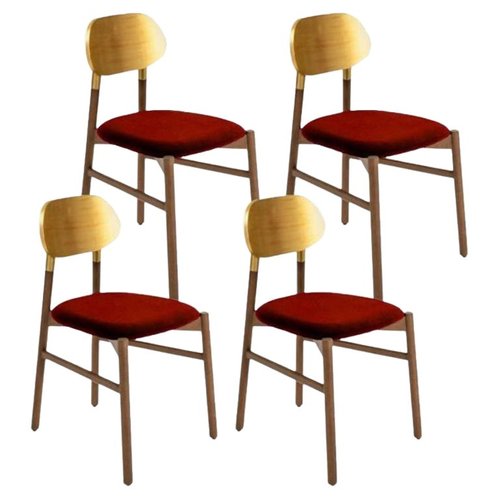Displayed against a plain white background, the image features four dining chairs arranged in a neat row. Each chair is supported by four slender metal legs, finished in a light brown hue that gives them a subtle rustic charm. Notably, these legs are interconnected by metal bars that link the front and back legs, enhancing the chairs' structural stability. The back legs extend upwards, culminating in a small, oval-shaped backrest crafted from light brown wood, which is smoothly rounded in the middle for added comfort. The seat of each chair is adorned with a red cushion, offering a vibrant pop of color; though not overly thick, it promises a comfortable seating experience. At the base of each leg, a discreet black tip caps the metal, likely designed to prevent floor scratches and ensure stability.